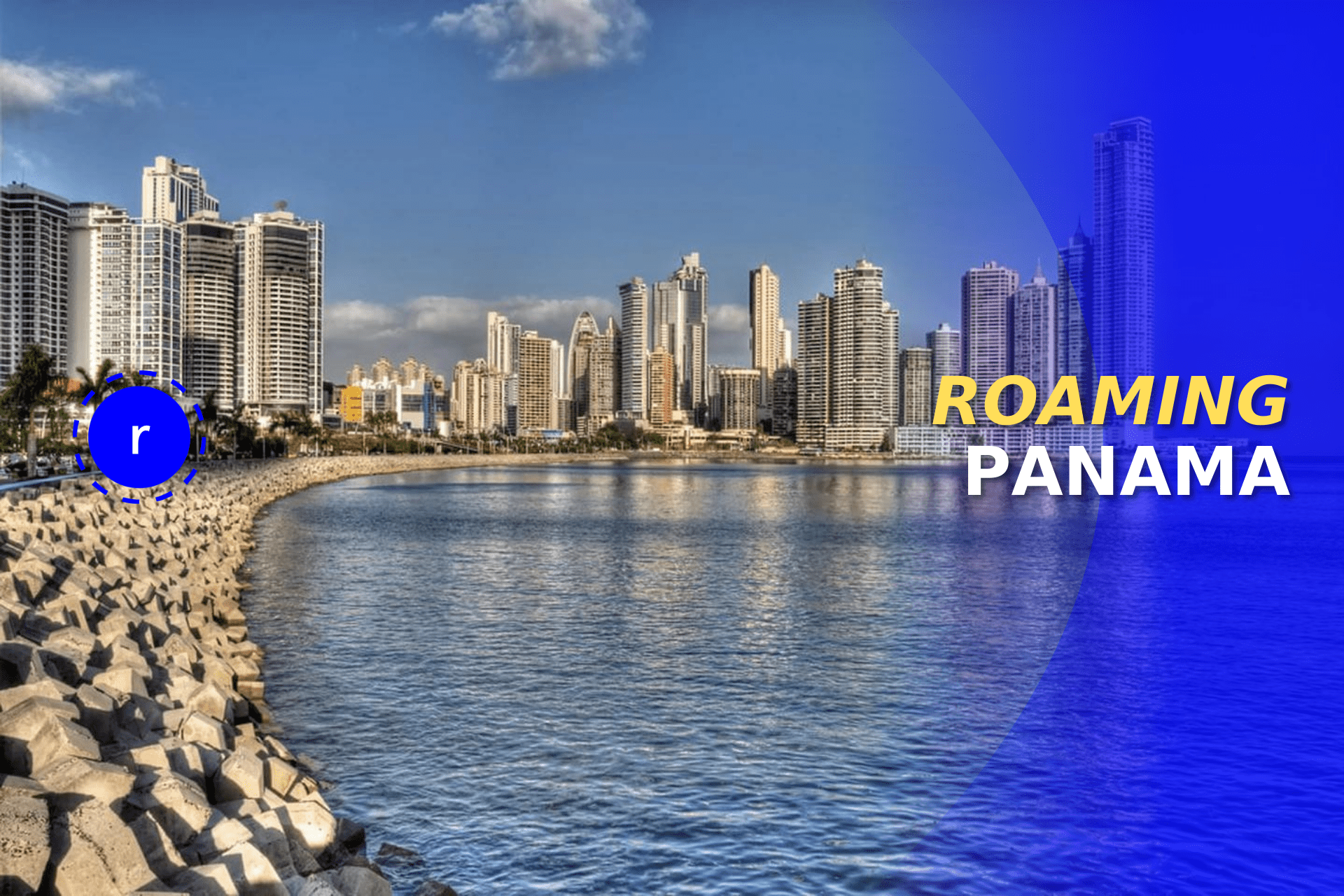This screenshot captures a stunning image of a downtown area along a riverfront, presumably in Panama, as indicated by the text "Roaming Panama." The scene is framed with beautiful rocks along the riverbank and features a logo with a white letter "R" inside a blue circle, accented by a dashed line border.

The sky is a vibrant blue with only a few picturesque clouds, enhancing the overall beauty of the image. Tall, majestic city buildings that resemble skyscrapers dominate the skyline, while palm trees add a touch of tropical charm to the foreground. The scene appears serene, with no noticeable people, suggesting that it was taken during a quieter time, possibly late evening. The sunlight bathes the buildings in a warm glow, reflecting splendidly off their surfaces.

The setting includes what looks like a boardwalk, inviting for leisurely strolls along the water. Given its captivating allure and clear details, this image could very well be part of an advertisement encouraging travelers to visit Panama and explore its urban and natural beauty.